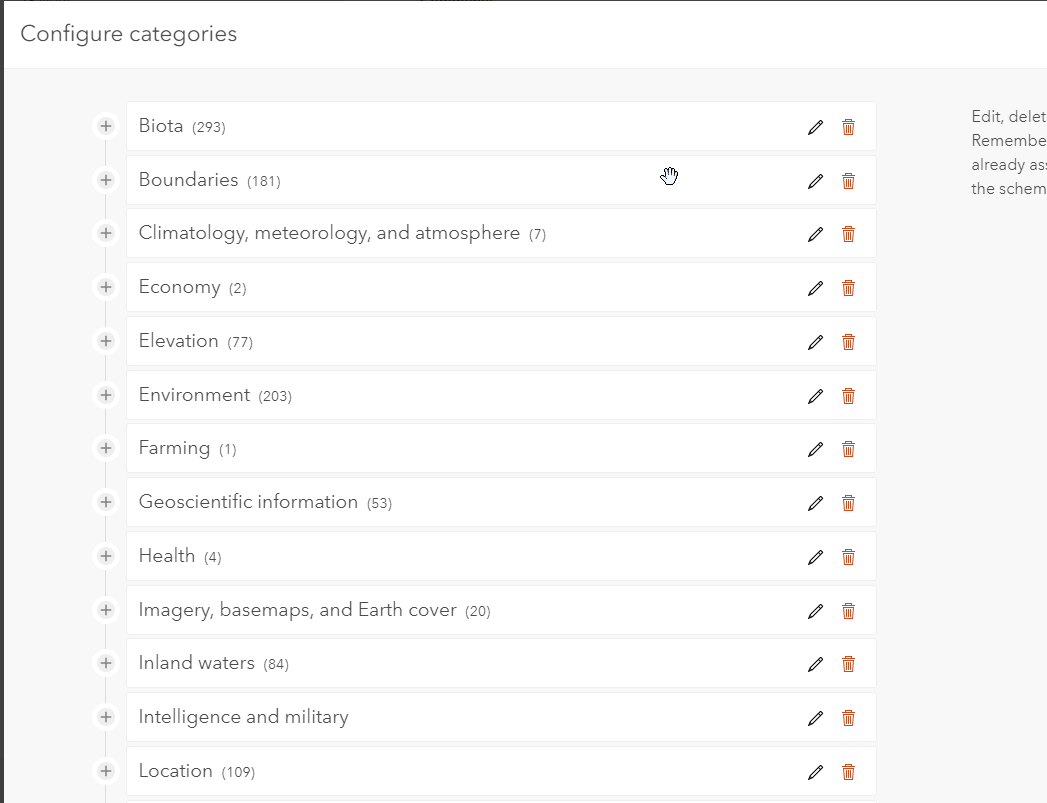The image showcases a text-based interface displaying a configuration screen for various categories. The background color is gray. Below is a detailed description of the elements present:

- At the top, the phrase "Configure Categories" is displayed prominently.
- Each category entry begins with a plus sign, followed by a white rectangular box containing the category's name, a count in parentheses, and two icons: a pencil for editing and a red garbage can for deleting.
- The categories listed are as follows:
  - **Biota (293)**
  - **Boundaries (181)**
  - **Climatology, Meteorology, and Atmosphere (7)**
  - **Economy (2)**
  - **Elevation (77)**
  - **Environment (203)**
  - **Farming (1)**
  - **Geoscientific Information (53)**
  - **Health (4)**
  - **Imagery, Base Maps, and Earth Cover (20)**
  - **Inland Waters (84)**
  - **Intelligence and Military**
  - **Location (109)**

- Each category includes the pencil and garbage can icons within their respective rectangular boxes, allowing for editing or deleting.
- A mouse hand icon is also visible, indicating the current cursor position.
- In the upper-right corner, there are options labeled "Edit," "Delete," and another unspecified option serving as part of the interface scheme.

The layout and design suggest a systematic approach to managing and organizing various data categories, with intuitive icons for modification and deletion, making it user-friendly and functional.